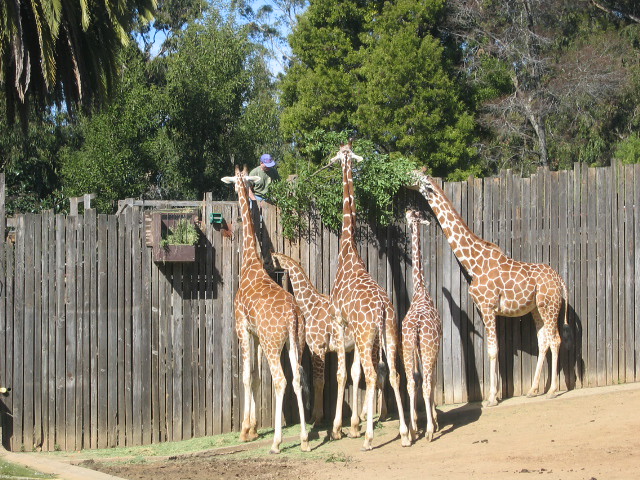This detailed photograph captures five giraffes in a zoo setting, standing amidst a dirty and grassy area in front of a weathered, gray wooden fence with vertical boards. Two adult giraffes, distinguished by their tall stature and brown circular spots on white bodies, are seen reaching over the fence, their faces buried in the foliage of a tree branch. A third adult giraffe is also indulging in the leaves, while another adult appears to be looking for food. Among them are two smaller, younger giraffes, one of which is too short to reach the top of the fence and appears curious rather than feeding. Behind the fence, diverse greenery includes palm trees and a lifeless, leafless tree. The scene features a person in a green t-shirt and a purple hat, possibly a zookeeper, who seems to be facilitating the feeding by holding the tree branch. Adjacent to the person’s position, a box feeder filled with leaves is attached to the fence, providing additional food for the giraffes.